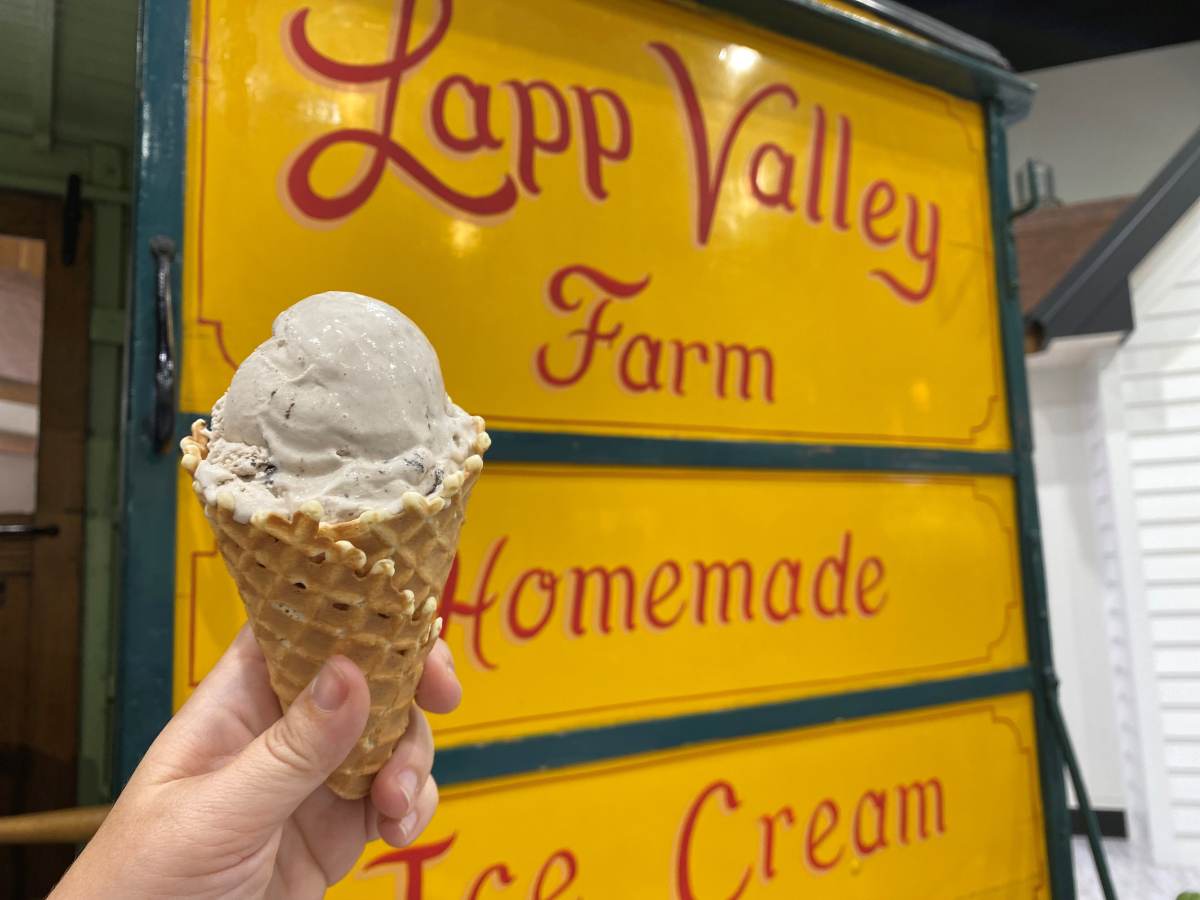The photograph features a brightly colored sign on the door of Lap Valley Farm, a business known for its homemade ice cream. The sign is constructed from three yellow slats with red, stylized cursive writing. The topmost slat spells out "Lap Valley Farm," followed by "Homemade" on the middle slat, and "Ice Cream" on the lowest one. The sign is mounted on a door that sports a green frame, suggesting a rustic, quaint setting. To the left of the door is a brown adjacent doorway, and to the right, the white siding of the building is visible, adorned with vertical slats, and capped with a shingled roof.

In front of the sign, a young person’s left hand prominently holds up a sugar cone with a single scoop of ice cream. The ice cream appears to be vanilla, perhaps with bits of cookie dough and chocolate chips embedded in the creamy white dessert. This hand, extending from the lower left of the frame, contrasts with the background, emphasizing the homey and inviting nature of the Lap Valley Farm ice cream experience. The overall composition effectively highlights the allure of a fresh, homemade ice cream treat against the backdrop of a charming, small-town business setting.